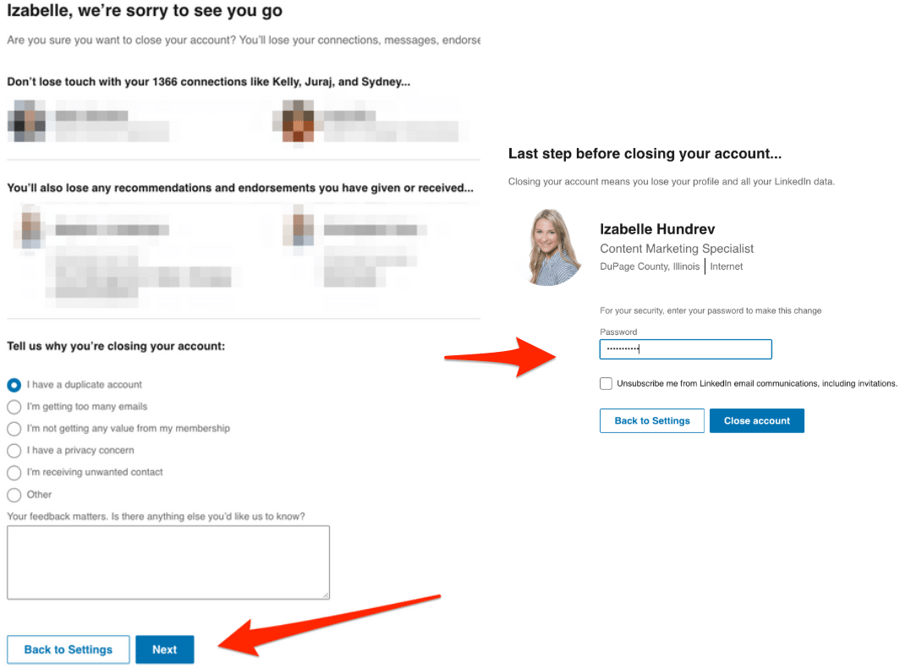The image depicts a user interface screen, likely from a social networking or professional connections platform, specifically for closing an account. In the upper left corner, a message reads, "Isabel, we're sorry to see you go," indicating the user's intent to leave the platform. Below this message, in a smaller gray font, a confirmation question asks, "Are you sure you want to close your account? You'll lose your connections, messages, and endorsements," though the text is partially cut off.

Beneath this, another message warns, "Don't lose touch with your 1366 connections, like Kelly, Jaraj, and Sidney." The interface is divided into two main sections. On the left side at the bottom, there are two buttons: "Back to settings" and "Next," situated below a section titled, "Tell us why you're closing your account."

On the right side, the heading reads, "Last step before closing your account." This section features the user's profile picture and prompts for enhanced security: "Enter your password to make this change." A password input box is visible, showing a password already entered.